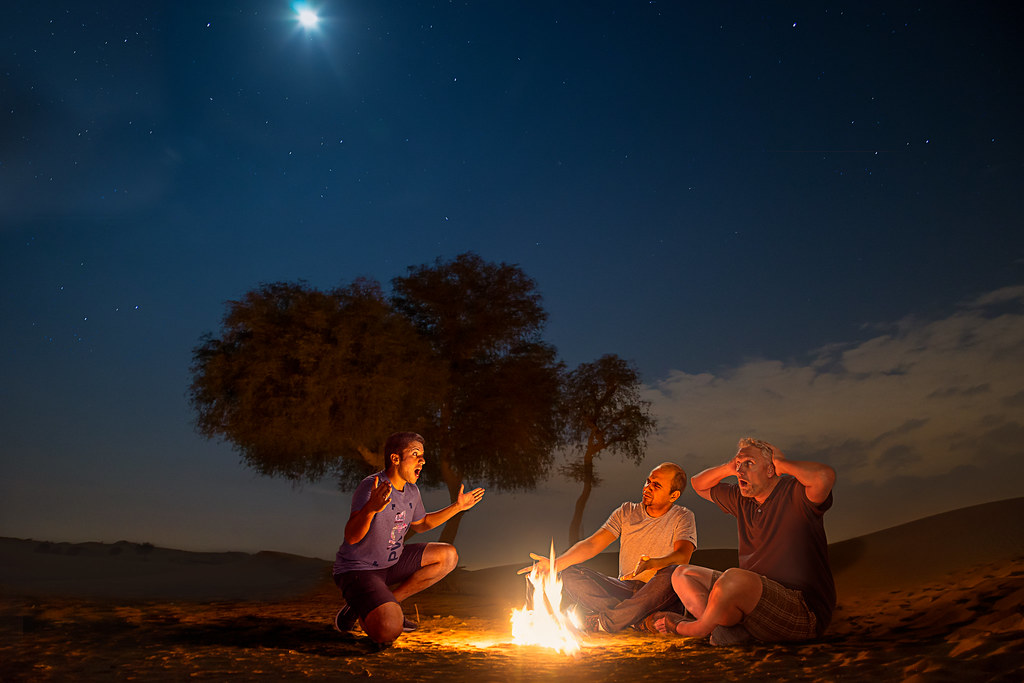The image depicts a nighttime scene in a remote, desert-like area under a dark blue sky dotted with stars and the glowing light of the moon, with light fluffy clouds visible. Three men form a circle around a crackling campfire, their faces illuminated by its flickering light. Two tall trees and one smaller tree stand silhouetted in the background. The man on the left is kneeling on one knee, animatedly telling a story with his arms wide open. He is dressed in a short sleeve blue t-shirt with some writing on it, black shorts, and sneakers. The middle man, who appears to be trying to warm his hands by the fire, is wearing a gray shirt and dark denim pants. The man on the right is clad in a black t-shirt and plaid shorts, sitting cross-legged with a shocked expression, his hands lifted near his head as if he can't believe what he's hearing. Despite the remote and serene setting, the men are visibly excited and engaged in their storytelling.